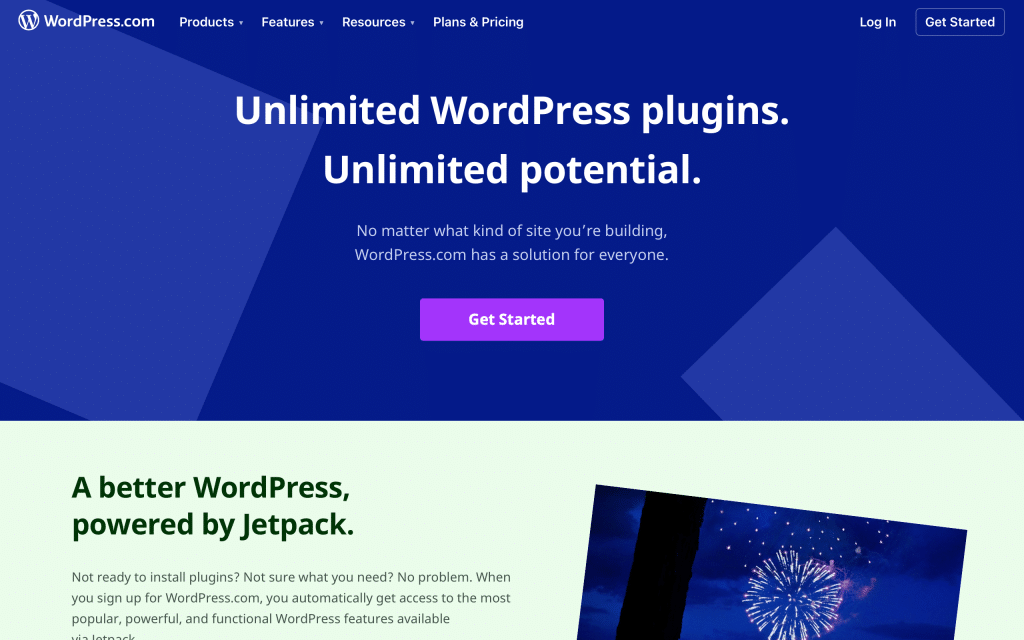The image captures a promotional segment of the WordPress website. 

In the upper left-hand corner, the iconic 'WordPress' logo is displayed in white. Adjacent to it are navigation links also in white: 'Products,' 'Features,' 'Resources,' 'Plans and Pricing.' The upper right-hand corner features 'Log In' and 'Get Started' in white text.

The background is a deep navy blue adorned with medium blue squares on either side. Dominating the center is a bold white headline that reads, "Unlimited WordPress plugins, unlimited potential." Below that, in smaller white text, it states, "No matter what kind of site you're building, WordPress.com has a solution for everyone."

A purple call-to-action button with white text, "Get Started," is positioned centrally beneath the headline. Below the blue section, a mint green rectangle sits, containing the text in dark green, "A better WordPress powered by Jetpack." The visible smaller green text further elaborates, "Not ready to install plugins, not sure what you need, no problem. When you sign up for WordPress.com, you automatically get access to the most popular, powerful, and functional WordPress features available."

The bottom portion of the screenshot is partially cut off but shows a dark blue rectangle featuring an image of fireworks extending beyond the visible area.